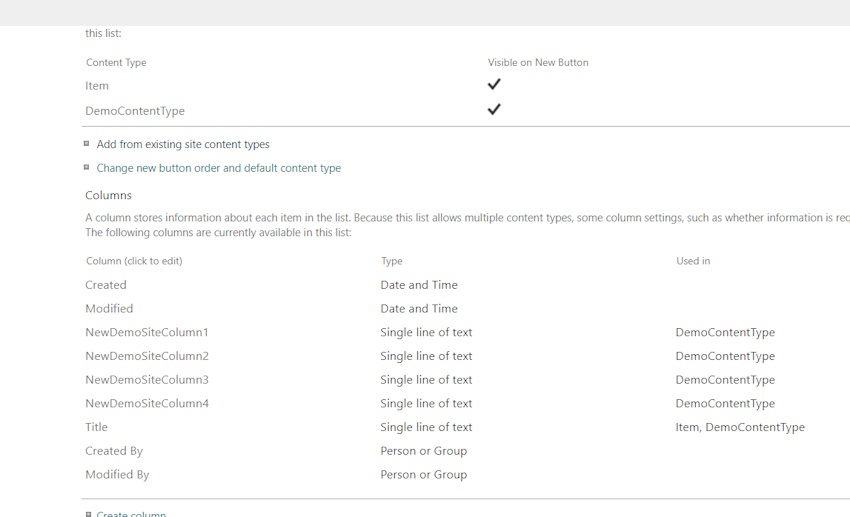A screenshot of a webpage titled "Content Type Settings". The page is filled with technical details and lists, making it challenging for a layperson to comprehend without context. At the top, there are categories such as "Content Type," "Visible on New Button," "Item," and "Demo Content Type," mentioned twice, emphasizing their importance or redundancy.

The page seems to be tailored for developers or users managing content types on a platform, possibly a content management system (CMS). It includes bullet points like "Add from existing site content types," "Change new button order," and "Default content type," which indicate options for managing various content types and their order of appearance.

A highlighted section titled "Columns" explains that this part stores information about each item on the list. Since the list allows multiple content types, it includes settings like whether specific information is required. The current columns listed include "Created" (with data type 'Date and Time'), "Modified" (also 'Date and Time'), and "New Demo Site Column 1" (with data type 'Single Line of Text'). 

The detailed nature of this page suggests it's designed for advanced users with knowledge of how to manage and configure content types in a web or CMS environment.